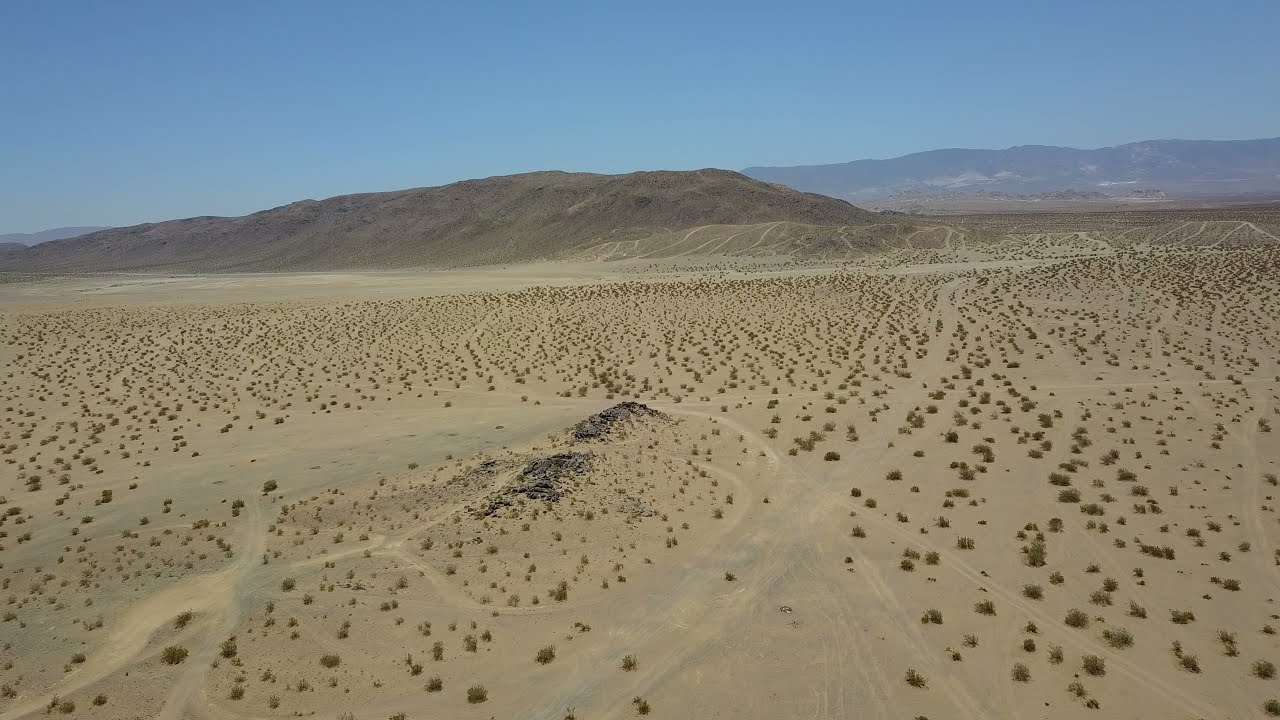In this image of a vast desert landscape, a clear blue sky fades from a lighter blue on the right to a darker blue on the left, stretching across the horizon without a single cloud in sight. The sandy desert floor, varying in hues from tan to brown with occasional patches of gray, is peppered with countless tiny green plants—likely a mix of cacti and brush—that blanket the terrain and extend all the way up the distant, rugged mountains. These mountains, while predominantly brown and rocky, have a slight blue hue due to the atmospheric distance. Sporadic rocks protrude from the sand in places, and subtle tracks or marks hint at the passage of a small vehicle. Despite the sparse vegetation, no signs of water, human presence, or structures disrupt the pristine isolation of this arid expanse.